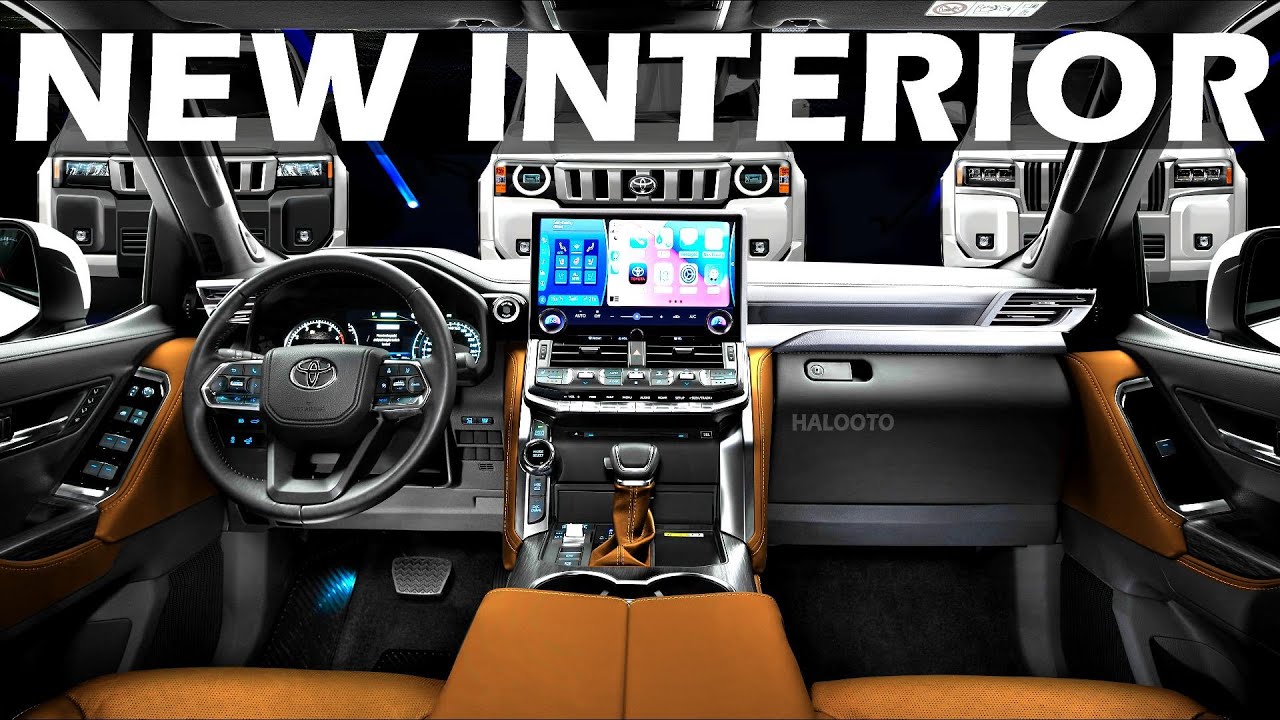The image captures the pristine and shiny interior of a car, emphasized by the bold white text at the top that reads "NEW INTERIOR." The focal point of the car's cabin includes light brown tan leather seats and black leather components like the steering wheel and glove box. The sleek dashboard hosts a prominent large screen, similar in size to an iPad, displaying various apps. Blue ambient lights illuminate the numerous buttons, adding to the modern aesthetics. The view seems to be from in front of the front seats, showcasing the front portions of the two seats, the steering wheel, and the central control system. Through the clear windshield and side windows, the exterior of three SUVs is visible, with two vehicles being white and one having a silvery black hue. Additionally, the car's interior door panel is gray, with the rest of the dashboard complementing this color scheme, highlighted by luxurious brown. The overall impression is one of sophistication and advanced design, creating a bright and inviting space.